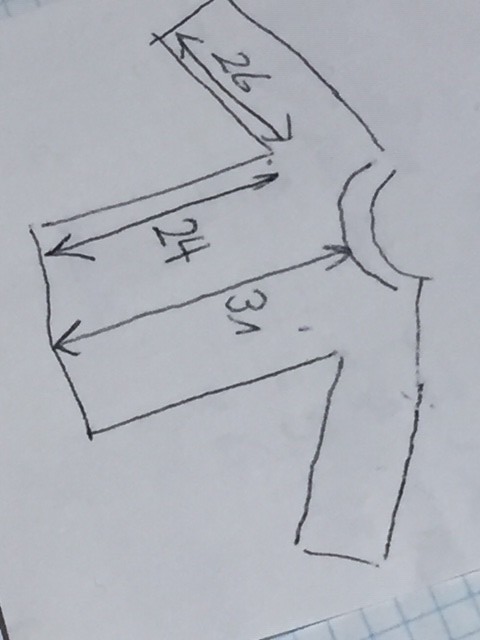This photo showcases a hand-drawn design of a long-sleeved top or shirt on white paper. The drawing is executed in either black pen or pencil. The paper is laid out on a fabric with thin blue lines forming a grid of small squares. The image itself is in portrait orientation, with the shirt's left sleeve extending toward the top of the picture and the right sleeve extending toward the bottom.

Specific measurements are noted directly onto the drawing:
- An arrow with two arrowheads marks the length from the cuff of the left sleeve to the underarm, indicating "26."
- Another double-headed arrow measures from the underarm to the bottom edge of the jersey, marked as "24."
- A third double-headed arrow aligns vertically from the bottom of the garment to its collar, noted as "30." However, the last digit is somewhat unclear due to poor handwriting, possibly resembling a "1."

The overall composition clearly illustrates the dimensions and layout of the garment design amidst a neatly patterned background.